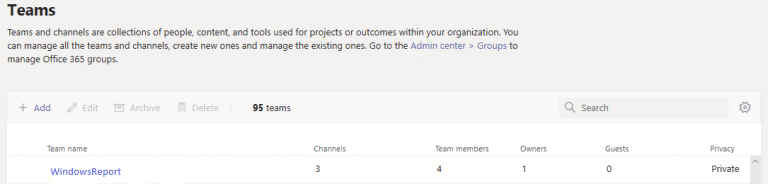The image displays a user interface for managing Microsoft Teams and Office 365 Groups. At the top, there's a gray rectangle labeled "Teams." The text explains that Teams and channels are collections of people, content, and tools used for projects or outcomes within an organization. Administrators can manage all the teams and channels, create new ones, and manage existing ones by navigating to the admin center. 

Highlighted in blue is the text "Go to the admin center," accompanied by a blue arrow pointing to the right, leading to the word "Groups" in blue. In black text, it says "to manage Office 365 groups." 

Beneath this section is a lighter tan rectangle that features a plus sign followed by the word "Add" in blue. Next to it, there's an icon resembling a pencil and the word "Edit" in gray. There's also a box labeled "Archive," and an indistinct label believed to read "Delete" next to it. The interface indicates "95 teams" are present. 

To the right of this, there's a magnifying glass icon next to the word "Search," and further right, there's a gear icon indicating settings. Below this, a white rectangle contains text that is too small and light to decipher. 

Under this section, the text "Window Reports" appears in blue, followed by numerical indicators at the bottom. Lastly, the word "Private" is displayed.